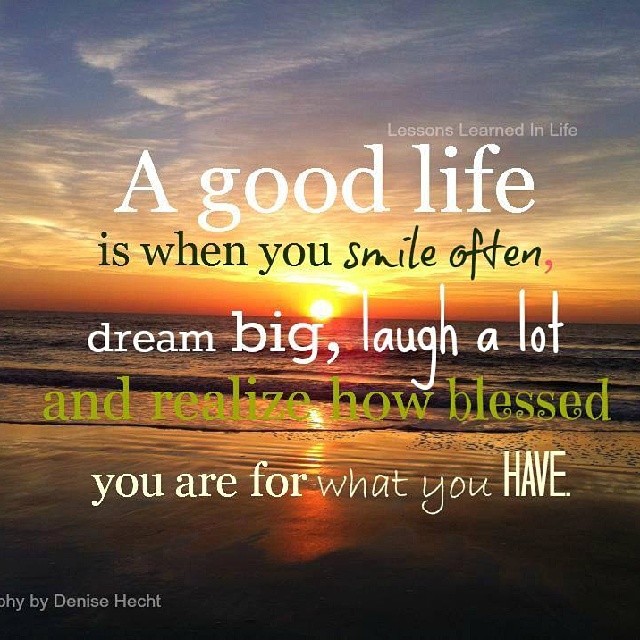A beautiful beach scene captures the sun just as it is about to sink below the horizon, bathing the landscape in warm golden and reddish hues. Wispy clouds stretch across the sky, fading into dark blue. In the foreground, gentle waves roll in towards the dark sand. Overlaying this stunning sunset are inspirational words: "Lessons learned in life" in small white print at the top right. Bold white letters declare, "A good life," followed by black letters, "is when you smile often." The next lines in white say, "dream big, laugh a lot," and in yellowish font, "and realize how blessed you are for what you have." At the bottom of the image, partially over the dark part of the beach, is the credit line, partially cut off but reading, "by Denise Hecht." This combination of captivating visuals and uplifting text creates a touching and motivational message.